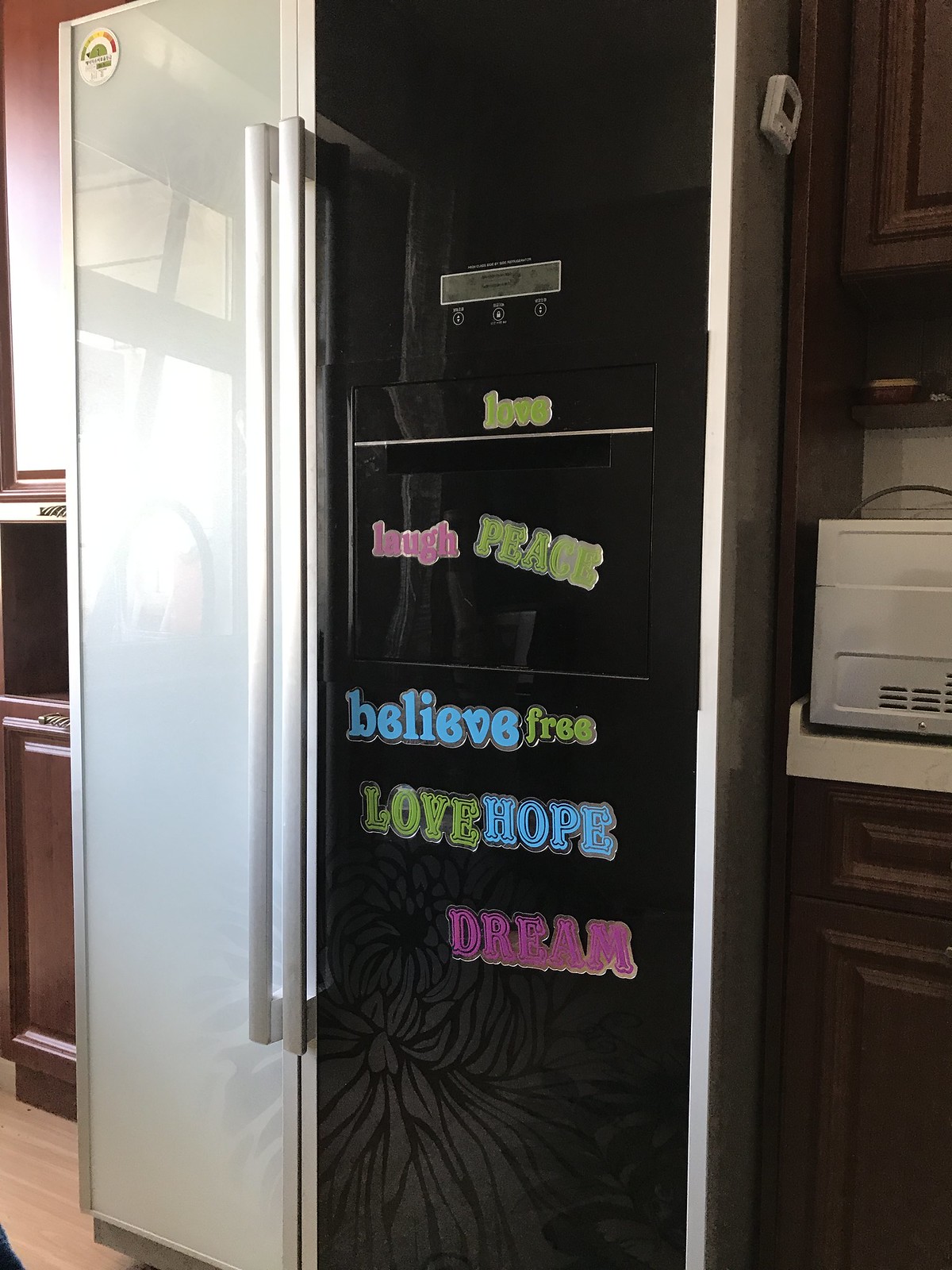This up-close photograph captures the center of a kitchen, featuring a side-by-side refrigerator with distinct black and white doors. The left door is white with a long silver handle and a circular brand logo at the top. The black right door also has a long silver handle and a gray-bordered digital display near the middle. The black door is adorned with various colorful word magnets: "love" in green, "peace" in green, "laugh" in pink, "believe" in blue, "free" in green, "hope" in blue, and "dream" in pink. Above these words, there is a line of unidentified green and pink words. To the right of the refrigerator, there are dark upper and lower cabinets with a white countertop, where a silver appliance, possibly a microwave, sits. A rectangular digital timer is magnetically attached to the silver side of the refrigerator. Brown cabinets frame the scene, enhancing the kitchen setting.